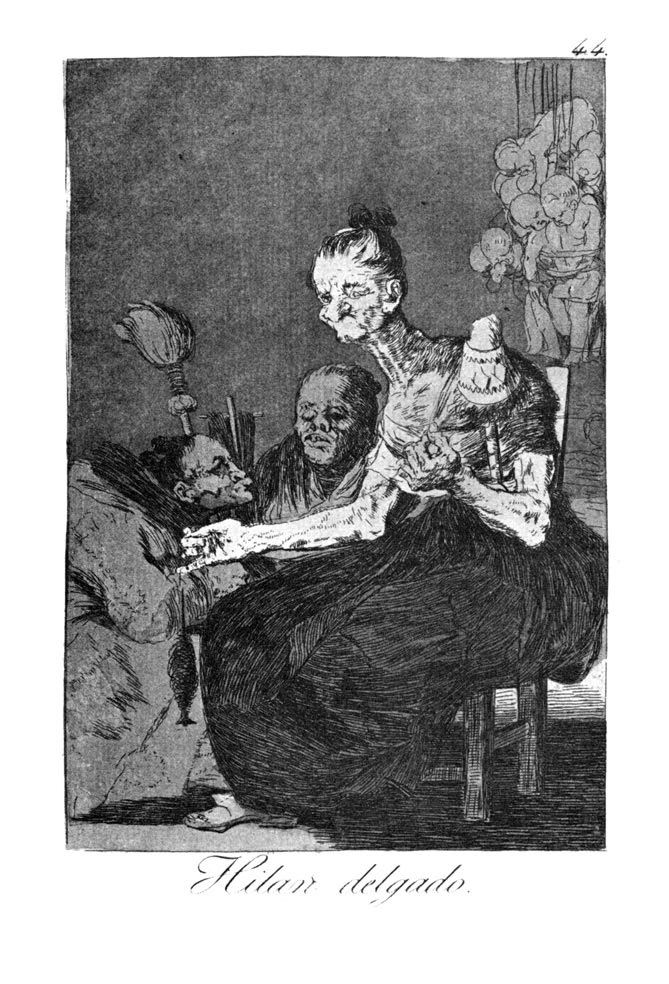A black and white drawing depicts a haunting scene with three grotesquely disfigured old women who appear to be witches. The central figure, seated in a wooden chair facing left, wears a long, dark dress. Her face is shriveled, with one eye closed and a long nose, and she clutches a fish on a line. Her hair is pulled back into a bun, and she displays unnaturally long and muscular arms. Behind her, two more crones, both appearing aged and stooped, are seen. One of them seems to be holding a broom aloft. The backdrop is dark gray, detailed with etching lines, adding to the eerie atmosphere. Disturbingly, naked babies or dolls are tied up and hanging from the upper right corner of the illustration. The entire composition is unsettling and surreal, capturing the macabre essence of a witch's lair. The cursive inscription "Hilan Delgado" is faintly visible beneath the drawing.